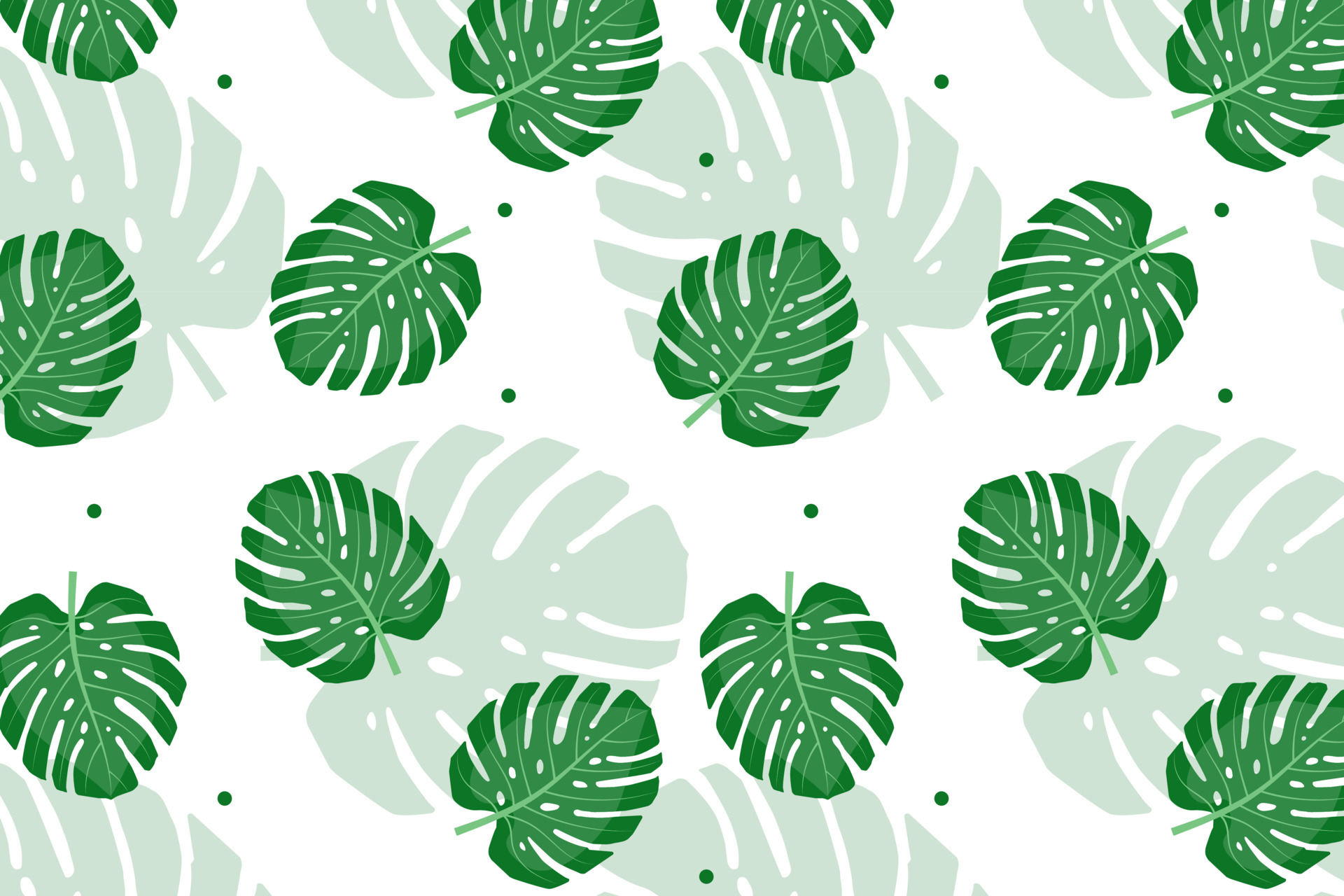This image is a detailed, digital pattern of palm fronds set against a white background, ideal for use in design applications such as wallpaper, clothing, desktop backgrounds, or art. In the foreground, there are numerous thick, green palm fronds, each intricately detailed and oriented in various directions, creating a dynamic visual effect. These foreground fronds are layered over larger, lighter-toned fronds in the background, which have a more muted, solid appearance and reduced detail, adding depth and contrast to the design. The image includes randomly distributed green dots that punctuate the white space, further enhancing the pattern. The overall composition has a rectangular, landscape orientation, and the repetitive nature of the palm fronds gives it a cohesive and harmonious look, suitable for a variety of decorative purposes.